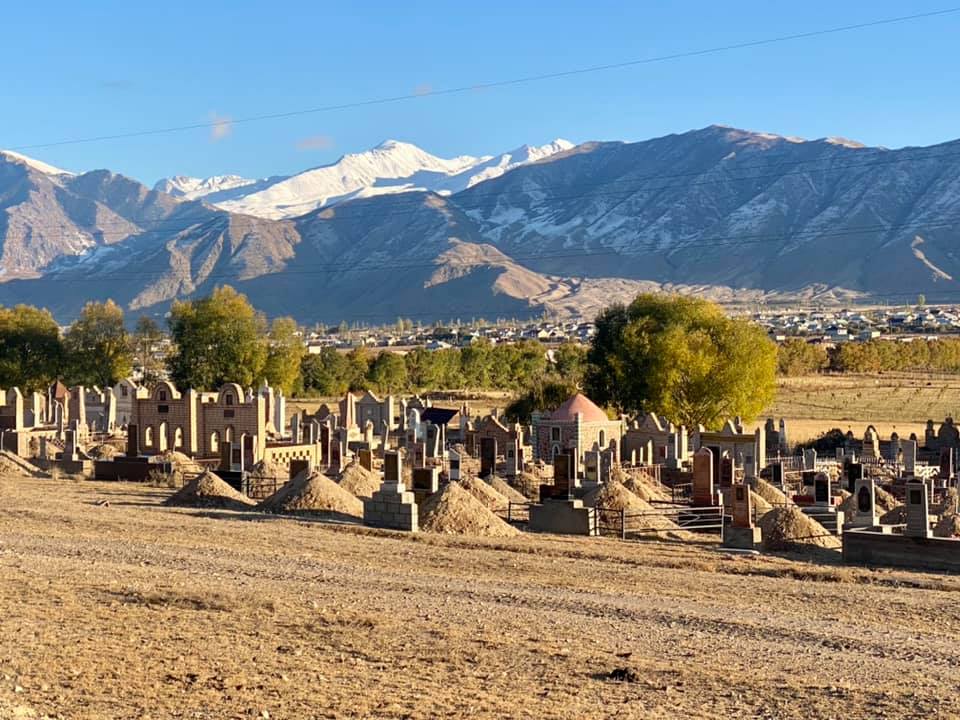This outdoor image captures a clear, blue sky with two small clouds and a power line crossing overhead. In the background, a stunning mountain range showcases its varied hues and snow coverage. The most distant peaks are snow-capped, contrasting with the darker gray and lightly snow-dusted mountains closer to the viewer. Below the mountains lies a bustling cityscape, accompanied by an orchard-like tree line. In the foreground, there's an intriguing, miniature kingdom that appears to be a historical reenactment site, featuring half-open buildings, castles, and palaces amidst fences. Adjacent to this, the scene transitions into a graveyard, marked by numerous headstones and fresh mounds of dirt, adding a depth of history and contrast to the picturesque landscape.